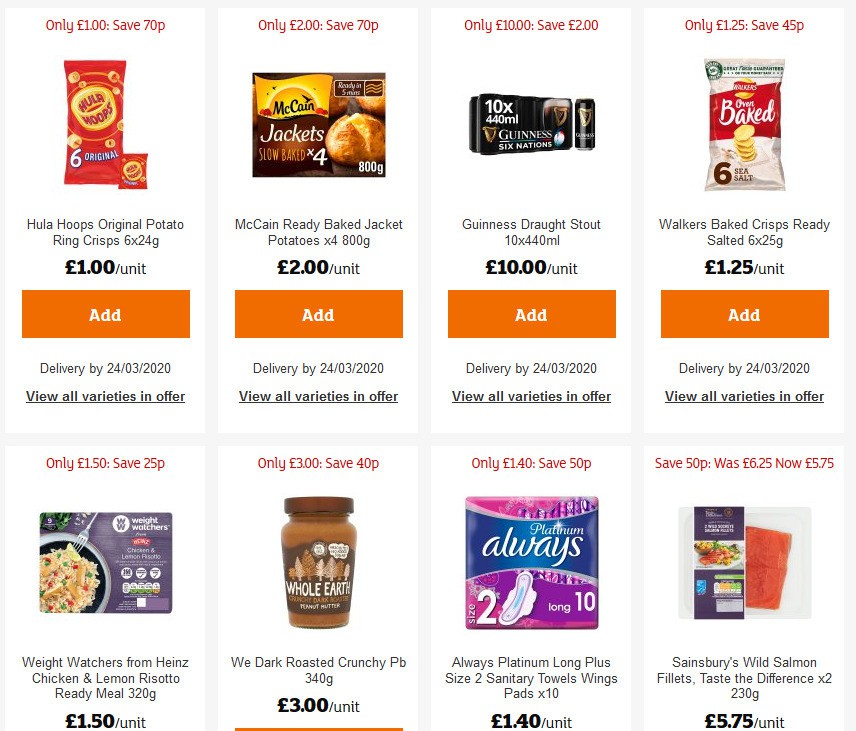The image depicts a detailed interface of a grocery shopping app showing various products available for addition to the cart. 

At the top of the app, there is a section labeled "Only $1.00 - Save 70p," featuring multiple snack items. The first product is a pack of Hula Hoops Original Potato Rings, priced at $1.00 per unit. There is an "Add" button next to each product to add them to the cart. The app also offers the option to view a variety of these products. 

Next on the list is McCain Ready-Baked Jacket Potatoes, available in a pack of four for $2.00 per unit, accompanied by an "Add" button. Following this is a unit of Guinness Draught Stout priced at $10.00, and a unit of Baked Crisps available for $1.25, also with corresponding "Add" buttons.

On the following row, a Weight Watchers from Heinz Chicken and Lemon meal is displayed with a picture of the TV dinner box above it. Currently priced at $1.50, it shows a savings of 25 cents from its original price of $1.75. However, the "Add" button for this product is partially cut off.

Further down, there is a product labeled "Dark Roasted Crunch" priced at $3.00 per unit, Platinum undergarments priced at $1.40, and Wild Salmon Fillets listed at $5.75. Each item retains an "Add" button for convenient shopping.

In summary, the app offers a variety of grocery items with prices and available discounts clearly displayed, facilitating an easy and efficient shopping experience.